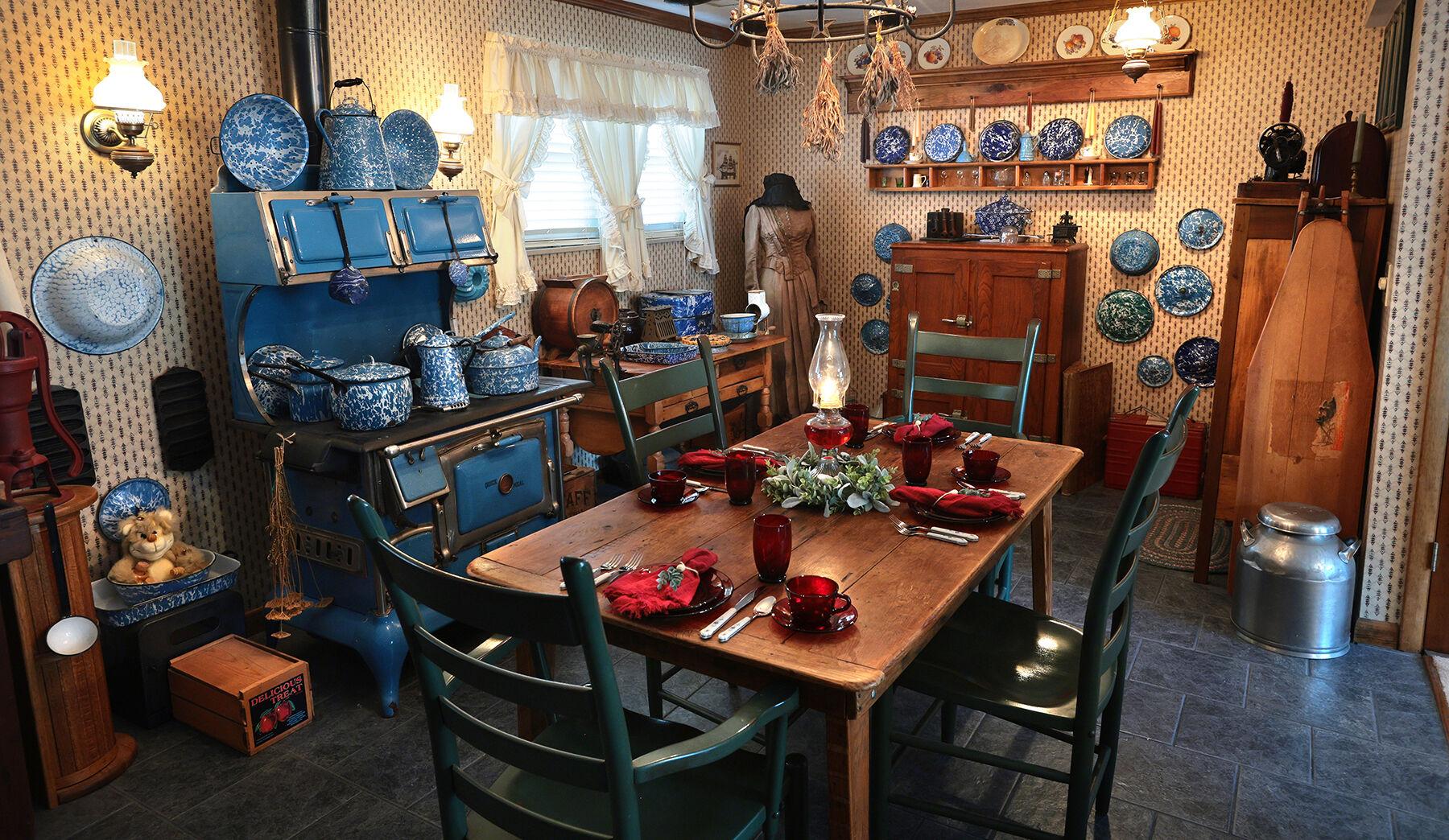The image depicts a nostalgic kitchen and dining room, reminiscent of the early 1900s. Dominating the center is a rectangular wooden table, framed by four black wooden chairs, one at each end, and another pair along the sides. The table is elegantly set with black plates atop a red tablecloth, complete with utensils neatly arranged. A flower pot and a slender vase add charm to the table's centerpiece. To the left, an old-school oven with a characteristic black pipe extends upwards and is adorned with blue pots and pans, enhancing the vintage aesthetic. The sink on the right features a wooden design, complimenting the rustic theme.

The kitchen's back wall is lined with brown wooden shelves holding blue and white plates, with additional blue and white decor mounted on the wall itself. A window with white curtains is nestled in the back left corner, allowing light to filter in. There is a stainless metal milk jug and a wooden ironing board contributing to the period’s authenticity. An intriguing touch is the hand pump for water, a common feature of the era. Completing the scene is a mannequin dressed in period attire, adding a lifelike element to the space. The wallpaper is white with a black pattern, enhancing the room's historical ambiance, echoed by the wooden apple crates scattered around.